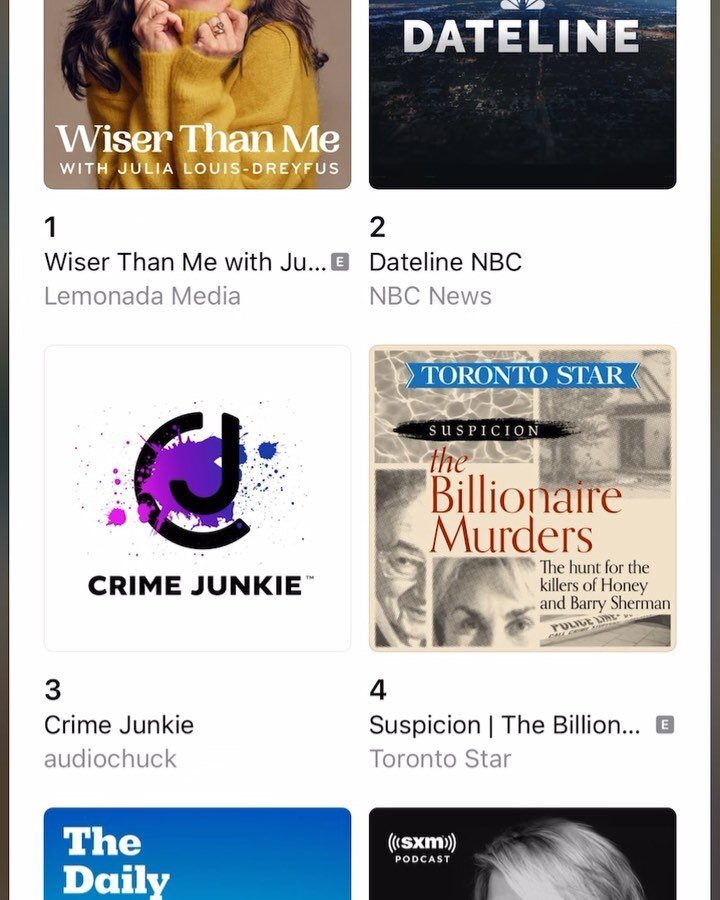The image depicts a screenshot of a digital interface, likely a website or app, that showcases a selection of popular podcasts. It features a ranked list with four clearly visible podcast covers, each associated with a numbered position from 1 to 4, and partially visible covers for two additional podcasts at the bottom. 

In the top-left corner, occupying the number one spot, is the podcast "Wiser Than Me with Julia Louis-Dreyfus." Adjacent to it is the second podcast, "Dateline NBC" by NBC News. Position three is held by "Crime Junkie" by Audio Chuck, and the fourth spot features "Suspicion: The Billionaire Murders - The Hunt for the Killers of Honey and Barry Sherman" by the Toronto Star.

At the bottom of the image, though partially cut off, two more podcasts are visible: "The Daily" and an unidentified podcast labeled as an SXM podcast. The background color of the interface is a clean and simple white, making the podcast covers and titles stand out prominently.